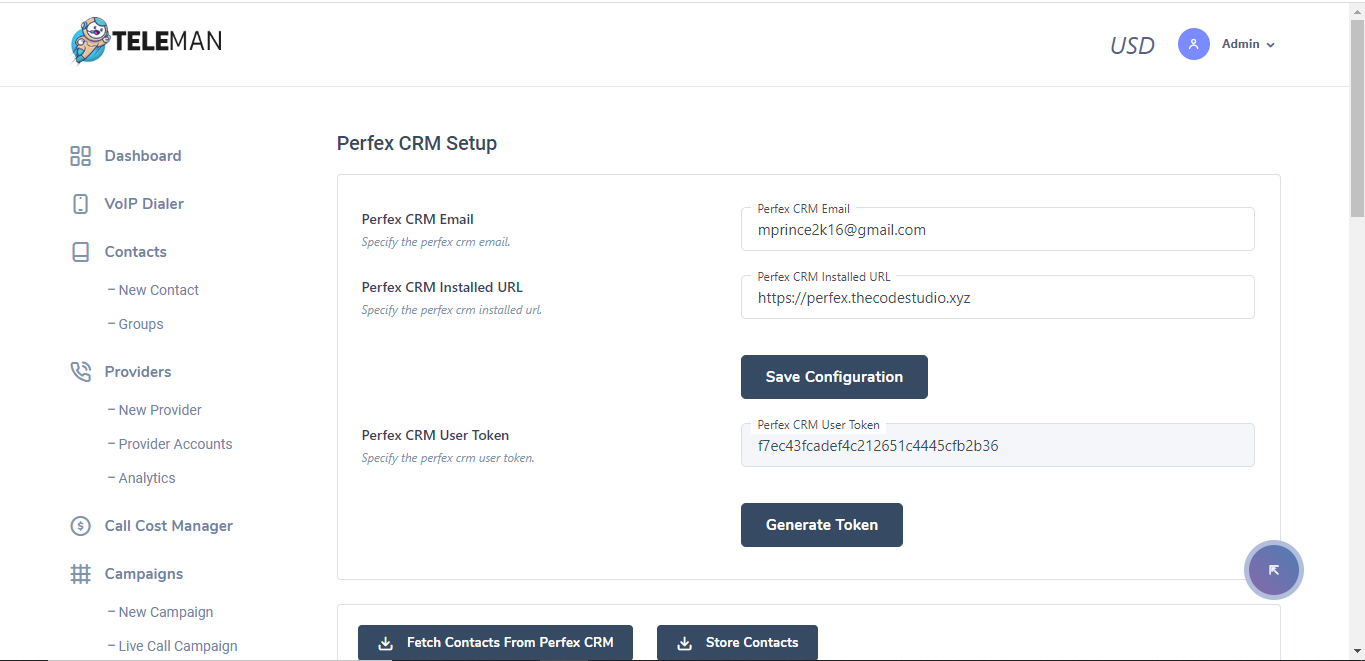Here is a cleaned-up and detailed descriptive caption for the image:

---

The image depicts a computer screen with a user interface on a white background. At the upper left corner, there is a logo that reads "Teleman," with "T-E-L-E" in bold. Next to the text, there is an icon of a small man in a yellow suit inside a blue circle.

In the upper right corner, there is an admin button accompanied by a dropdown menu for currency selection, defaulted to USD. A scrollbar is positioned along the right edge of the screen, fully scrolled to the top.

The interface is divided into several sections by light gray borders. The left side features a navigation menu with options including Dashboard, Contacts, and Providers.

The central portion of the screen prominently displays the text "Perform Perfect CRM Setup" inside a light gray rectangular outline. Below this heading, the section is divided into two columns.

In the right column, there are two rectangular blue buttons with white text, labeled "Save Configuration" and "Generate Token." Below these buttons, there are two additional buttons labeled "Fetch Contacts" and "Store Contacts."

---

This caption provides a comprehensive and organized description of the image, making it easier for readers to visualize the interface.